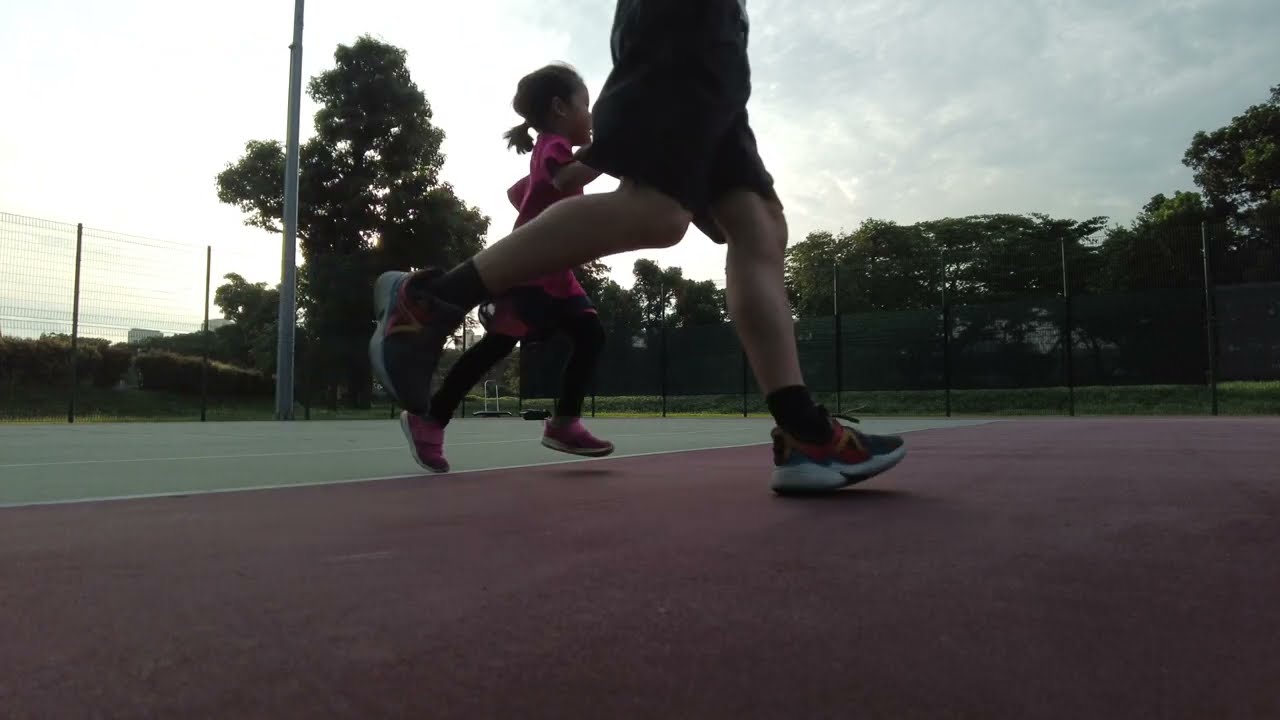In the image of an outdoor tennis court, a large adult male, visible only from the waist down, is in mid-stride, running towards the right. He is dressed in a gray t-shirt, black shorts, and brightly colored red, yellow, and black tennis shoes with white soles. Next to him, running alongside and slightly behind, is a young girl with her black hair tied in a ponytail. She wears a pink shirt, black pants, and pink shoes with white bottoms. The young girl's feet are off the ground, capturing the action of their run. They are on a tennis court, which features a distinctive red and green color scheme. A green fence with green and white posts surrounds the court, and to the left side of the image stands a silver pole supporting a light. The background shows a cluster of green trees and a gray sky.